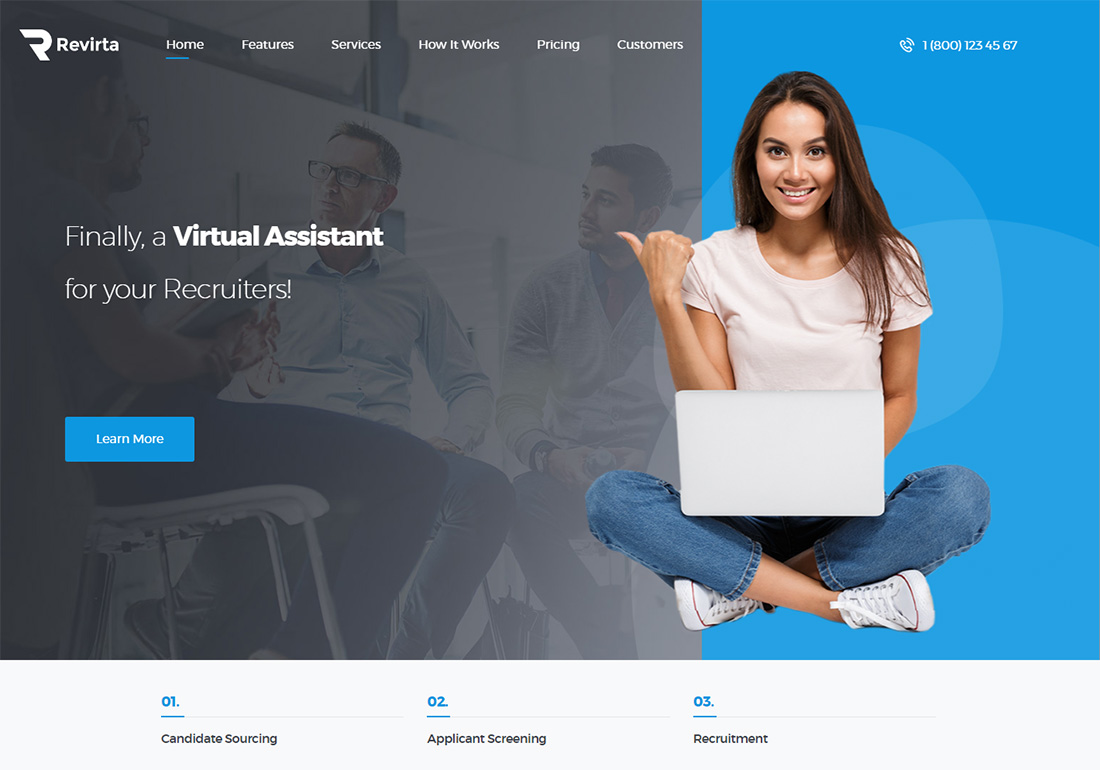The web page is an advertisement for ReVirta, a virtual assistant service company. The ReVirta logo features an R with the left leg cut off. The navigation bar at the top includes options such as Home, Features, Services, How It Works, Pricing, and Customers, with the Home button highlighted with a blue underline, indicating the current section.

The design of the page is divided into thirds. Two-thirds of the page on the left side has a light gray background showing an image of people collaborating closely, suggesting a productive work environment. Overlaying this image is a prominent text that reads, "Finally, a virtual assistant for your recruiters," accompanied by a blue clickable box that says "Learn more."

The remaining third of the page on the right side features a blue background with an image of a young girl with straight brown hair, wearing a white t-shirt, jeans, and Converse shoes. She is sitting cross-legged with a laptop on her lap—depicted as a simple rectangle. Her right arm extends, thumb pointing towards the left to the gray area with collaborating people, possibly highlighting the connection to the virtual assistant service. At the top right corner, there's an 800 number for potential customers to call and inquire about purchasing a virtual assistant.